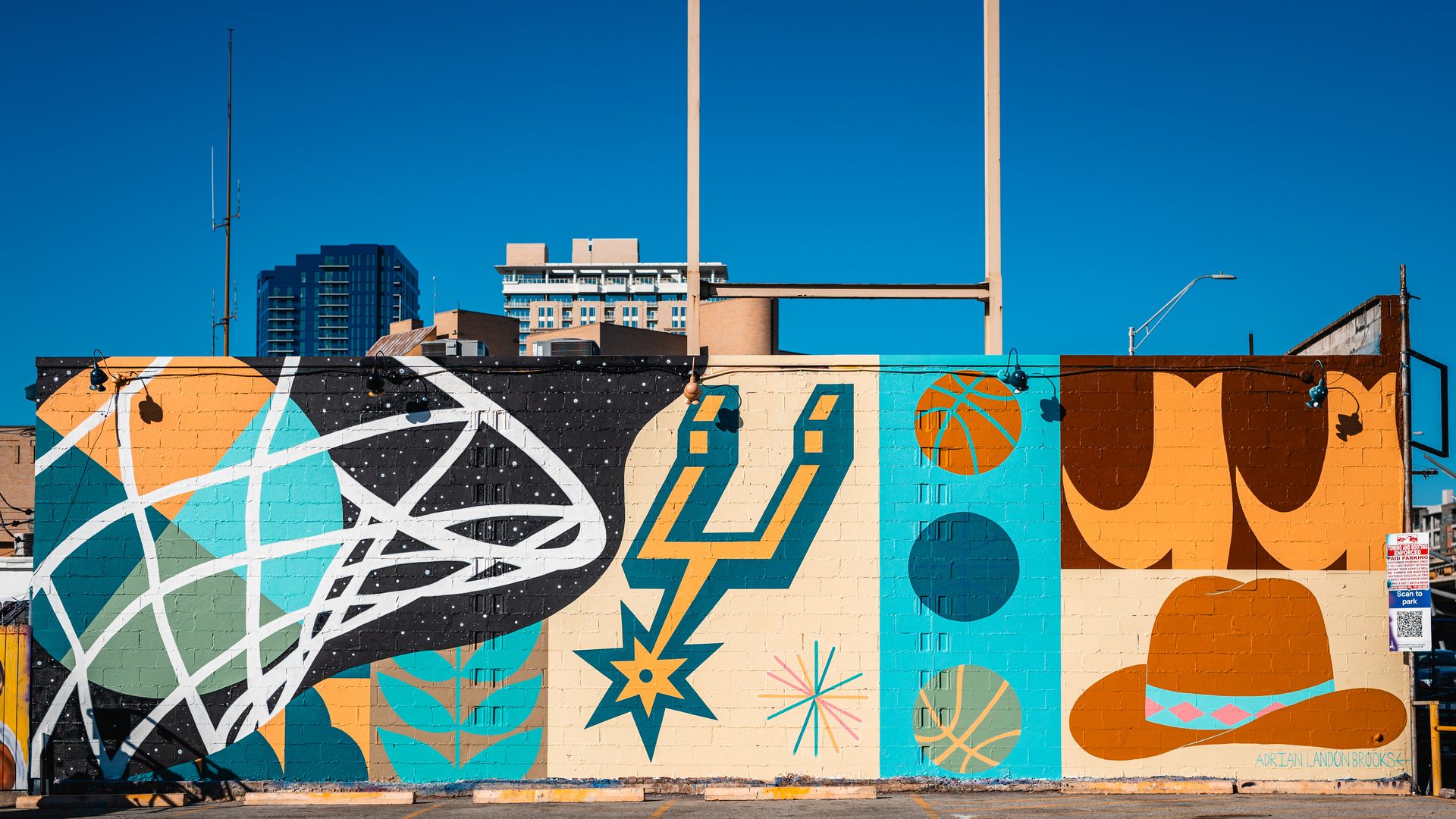The photograph captures a vibrant outdoor scene featuring a detailed mural on a tall brick wall, set against a clear blue sky. The mural, rich with beige, blue, brown, orange, and yellow hues, is primarily basketball-themed. On the left side, a black background showcases a white basketball net with a ball going through it, and a starry night motif. Adjacent to this, the San Antonio Spurs logo is prominently displayed in white, yellow, and blue. Further to the right, abstract art blends into a whimsical design featuring cowboy boots and a hat. Below, the mural extends to a section with three balls—a basketball, a blue ball, and possibly another sports ball—over a blue bar. In the background, an antenna and multi-storied buildings, including one painted blue, frame the scene, along with a light pole and a parking lot with stone rectangle markers and yellow lines visible on the pavement. This lively intersection of sports, art, and urban architecture captures the essence of an inner-city environment.